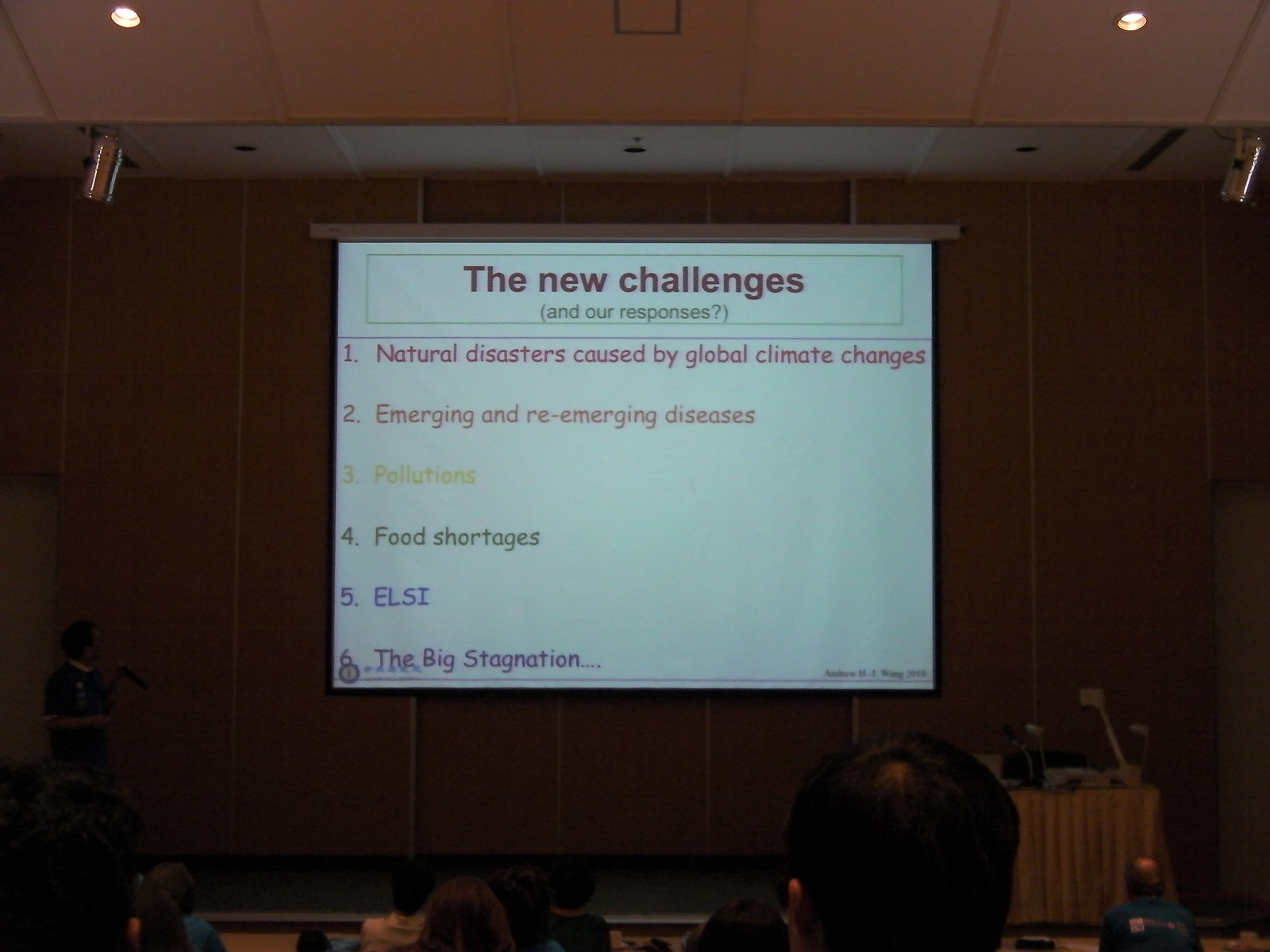This photograph captures a dimly lit lecture hall or conference room with a PowerPoint presentation projected on a large screen. The room is dark, possibly due to the camera's exposure settings or the minimal lighting, with only two ceiling lights turned on. The presentation screen prominently displays a slide titled "The New Challenges" with the subtitle in parentheses reading "and our responses". Below this title, a numbered list is presented in rainbow colors: 1. Natural Disasters Caused by Global Climate Changes (red), 2. Emerging and Re-emerging Diseases (orange), 3. Pollution (yellow), 4. Food Shortages (green), 5. ELSI (blue), and 6. The Big Stagnation (purple). There is a figure standing to the left of the projector screen, wearing a dark sweater over a white button-down shirt, and holding a microphone, seemingly presenting the content on the slide. In the foreground, the faint silhouettes of audience members' heads are visible, indicating the photo was taken from within the audience. The walls and ceiling tiles are hard to distinguish due to the low light, but there's possibly a podium or presentation table to the right of the screen. The overall scene suggests an academic or professional setting.